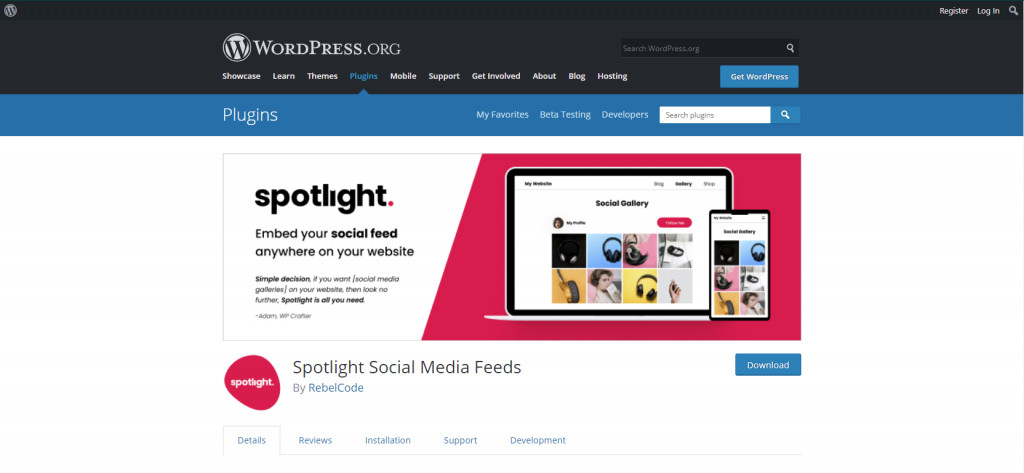The image depicts the WordPress.org homepage. At the top, there is a black navigation bar with "Login" and "Register" options on the top right, and a search bar positioned adjacent to these options. On the top left corner, the WordPress logo is prominently displayed.

Dominating the center of the page is a larger WordPress logo, with the text "WordPress.org" beneath it. Just below, a horizontal menu offers various options: "Showcase," "Learn," "Themes," "Plugins," "Mobile," "Support," "Get Involved," "About," "Blog," and "Hosting." On the far right, there's another search bar, accompanied by a blue button labeled "Get WordPress."

Further down, the page highlights a section that appears to be about plugins. It mentions titles like "My Favorite," "Beta Testing," and "Developers." One of the featured plugins is described under the heading "Spotlight: Embed your social feed anywhere on your website." The tagline suggests it’s a simple solution for integrating social media feeds into your site, stating, "If you want social media on your website, then look no further—Spotlight is all you need."

Accompanying this description is a blue "Download" button. The plugin is identified as "Spotlight Social Media Feeds" by RebelCode, with tabs for "Details," "Reviews," "Installation," "Support," and "Development."